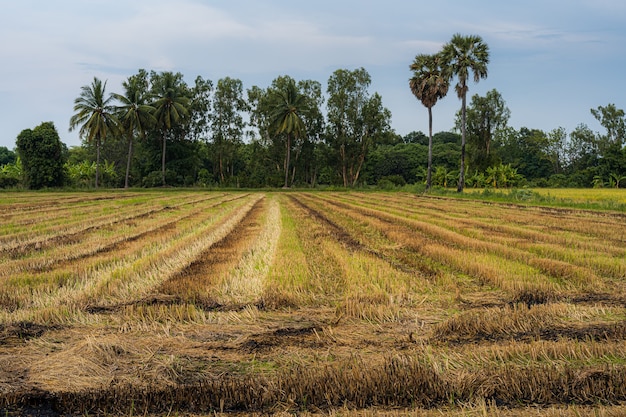The photograph showcases a vast open field plowed into distinct lines, with varying shades of tan, brown, and green creating a striped pattern across the straw-like ground. In the foreground, the field transitions from a dry, burnt appearance to patches of brownish dirt and grass. Encircling the field are numerous trees, prominently featuring palm trees interspersed with other taller greenish trees, and very dense bushes further in the background. The bright, sunny day bathes the landscape in natural light, highlighting the clear blue sky with slight cloud coverage. The scene is devoid of any people, animals, or vehicles, emphasizing the serene, expansive, and untouched nature of this farmland or possibly large lawn area.